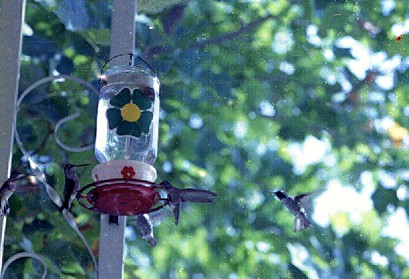In this outdoor daytime photograph, a clear glass hummingbird feeder with a red base hangs from a white or silver metal structure resembling an 'H' shape with intricate filigree detailing in the center. The feeder features small white porcelain cups adorned with red daisy-like flowers, and a larger green flower with a yellow center on its front. Surrounding the feeder, several hummingbirds are either perched or in mid-flight. One small black hummingbird with white and black bellies rests on the red base, while another hovers nearby with its wings blurred in motion. The background is dominated by a large, muted green tree with patches of sunlight filtering through the leaves, creating a serene and natural setting for this vibrant scene.